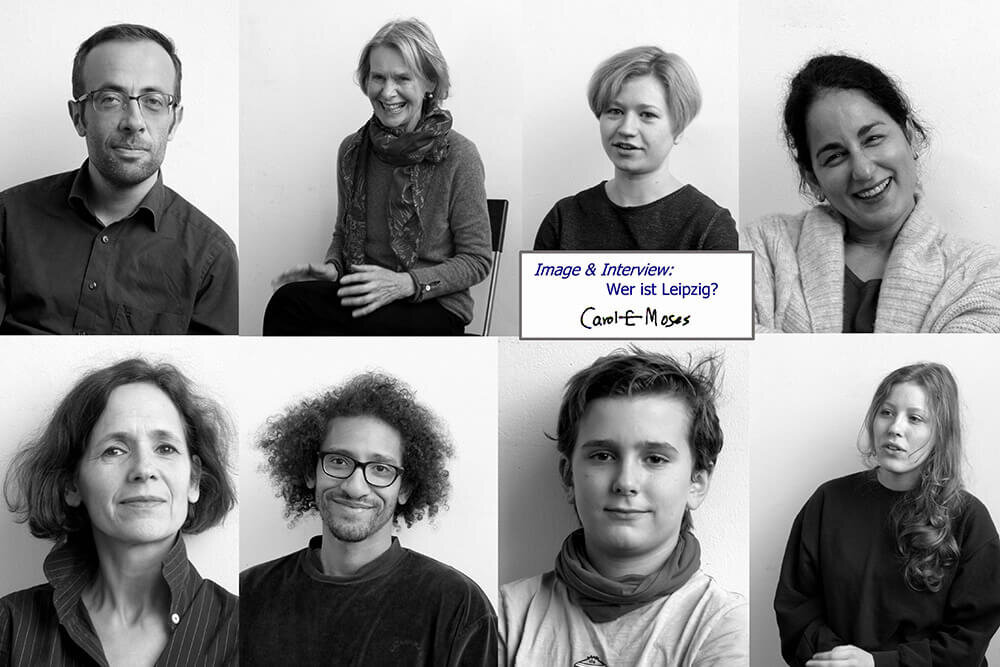The image displays eight black-and-white portraits arranged in two rows of four. At the center of the image, a white rectangle bears the text "Image and Interview" along with the German phrase "Wer ist Leipzig?" and the name Carol L. Moses in blue and black lettering. Each portrait features individual adults and children.

From left to right in the top row:
1. A man in his 30s with short brown hair, wearing glasses and a dark button-up shirt.
2. A slightly older woman, smiling, with short blonde hair, a cardigan, and a scarf around her neck.
3. A younger woman with short blonde hair, captured from head to just below the neck, wearing a black top.
4. Another woman, smiling with her head tilted, sporting dark hair and a light cardigan.

From left to right in the bottom row:
1. A middle-aged woman with light skin, short dark hair, and a collared shirt looking directly at the camera.
2. An ethnic man with very curly hair, black-rimmed glasses, and a dark sweater.
3. An adolescent boy with short brown hair, wearing a t-shirt and a scarf, looking at the camera.
4. A young adult woman with long brown hair, wearing a black sweatshirt and looking slightly off-camera.

The only colors in the image are shades of black, white, gray, and dark blue.